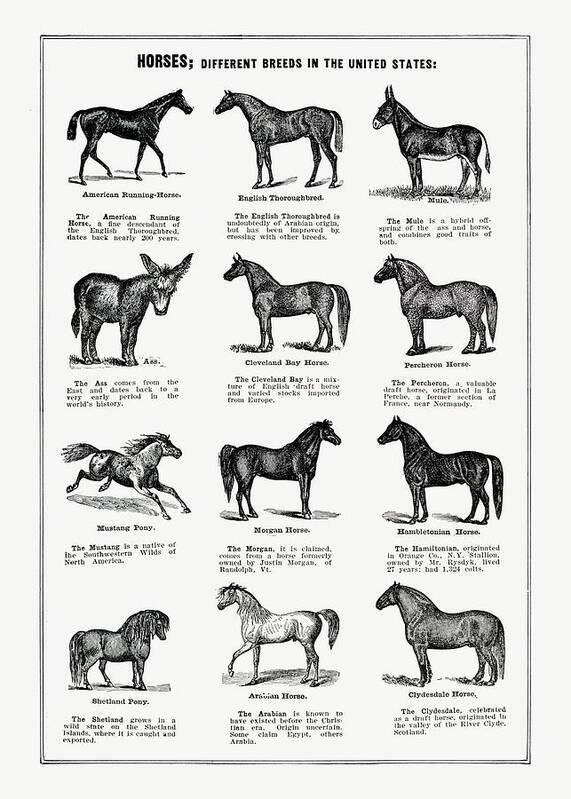The poster, titled "Horses: Different Breeds in the United States," is an illustration displayed within a vertical rectangular shape, bordered by a light or off-white color and outlined in dark gray or black. Showcasing a total of twelve different horse breeds—three across and four down—the poster is arranged into neat rows and columns. 

Each horse illustration, rendered in shades of black, white, and gray, is labeled with the breed name and accompanied by a small paragraph of detailed information, although the text is too small to read clearly. The top row features the American Running Horse, English Thoroughbred, and a Mule. The second row includes the Ass, Cleveland Bay Horse, and Pembroke Horse. In the third row, the Mustang Pony, Morgan Horse, and Hamilton Horse are displayed. Finally, the bottom row consists of the Shetland Pony, Arabian Horse, and Clydesdale Horse. 

This monochromatic poster not only serves as a visual guide to various horse breeds in the United States but also provides brief descriptions beneath each illustration, making it an informative and detailed piece despite the small and hard-to-read text.